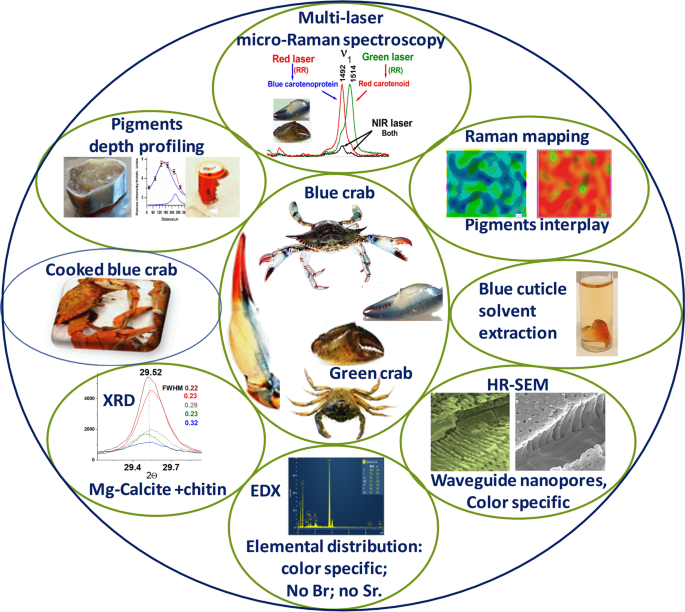The image is a detailed scientific diagram encapsulated within a large blue circle. Inside this blue circle, various green circles each contain specific research topics and corresponding images. At the top, the green circle is labeled "Multilaser Microraman Spectroscopy," showing a graph with varying lines and lasers. Moving clockwise to the top right, another green circle labeled "Raman Mapping Pigments Interplay" features blue and red images. Continuing clockwise, the next circle is labeled "Blue Cuticle Solvent Extraction," accompanied by an image of a tube. Below that, the circle reads "HRSEM Waveguide Nanopores, Color Specific," featuring images of nanopores. At the bottom, there is a circle labeled "EDX Elemental Distribution, Color Specific, no BR, no SR," displaying a relevant graph. To the bottom left, the circle is marked "MG Calcite plus Chitin," accompanied by another graph. Moving upward, the next circle labeled "Cooked Blue Crab" depicts an image of a cooked crab. Above this, a circle titled "Pigments Depth Profiling" shows a profiling graph of pigments. Centrally located within this diagram is a large green circle containing images of "Blue Crab and Green Crab." Each of these elements provides a comprehensive overview of the various scientific methods and research topics discussed in the study.